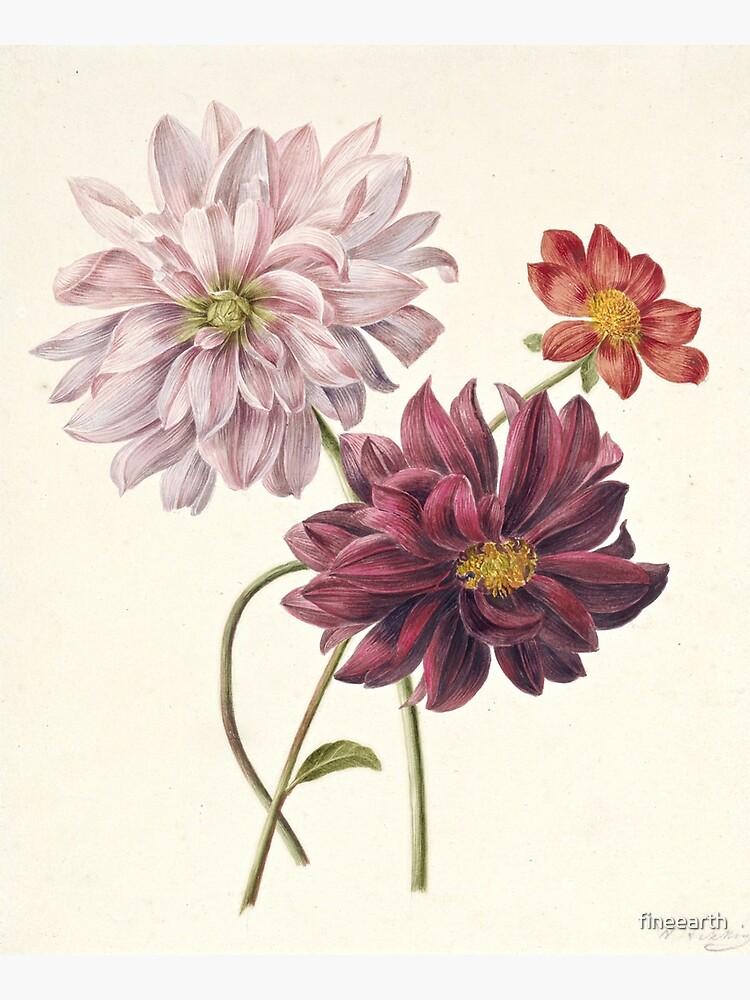This image features a vintage-style print of three meticulously illustrated flowers, set against an off-white, yellowed cream background. Each flower, complete with stems, is drawn with intricate detail and vibrant hues that range across a cohesive pink, red, and maroon color palette. The top left flower showcases an abundance of petals in multiple shades of pink and white, with a light green center. To its right is a smaller bloom, characterized by light red petals that deepen towards the tips, transitioning to a darker red at the center. The flower at the bottom is the largest, with densely packed, deep maroon petals accented with almost black shadows and a yellow center. At the bottom right corner of the piece, the text "vintage wall art" subtly denotes its classic design.